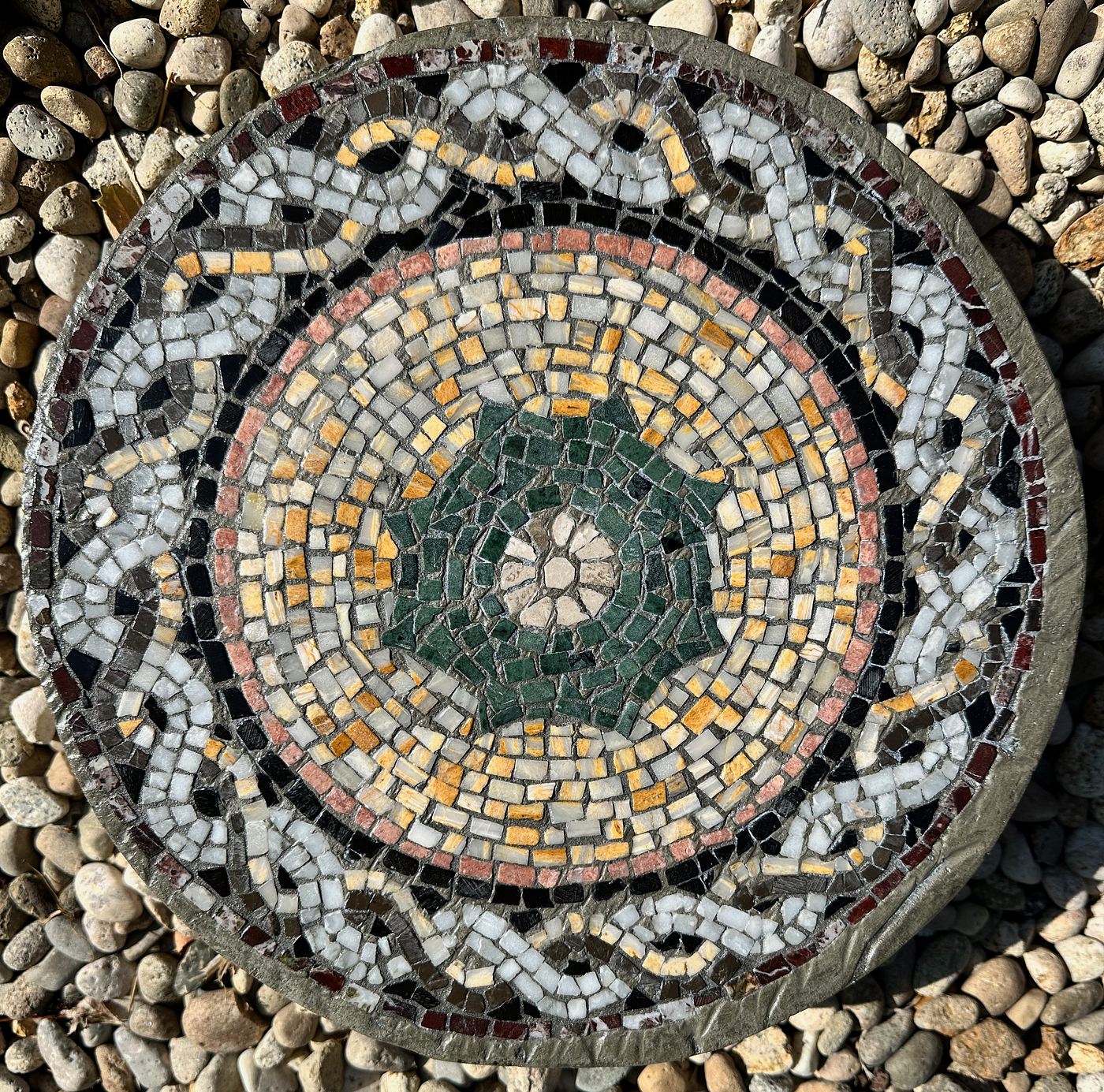The image depicts a large, circular mosaic stepping stone set amidst a collection of small, multicolored rocks, possibly in an outdoor backyard river wash. The photograph, taken during the daylight, shows the stone casting a shadow to the right, indicating a bright, sunny day. The stepping stone features a detailed, intricate design composed of multiple concentric circles. The outermost rim is gray, transitioning into a vibrant rainbow of blue, yellow, and gray, with a stripe of black mosaic tiles. A section of intertwining, snake-like patterns in blue and yellow follows inward, leading to a red circle that contains six smaller circles. At its core, the mosaic reveals a star pattern rendered in dark green, radiating from a central white point. The entire piece showcases an impressive array of colors and intricate craftsmanship, adding a beautiful, decorative touch to the surrounding landscape of diverse, small stones in shades of gray, brown, blue, and green.